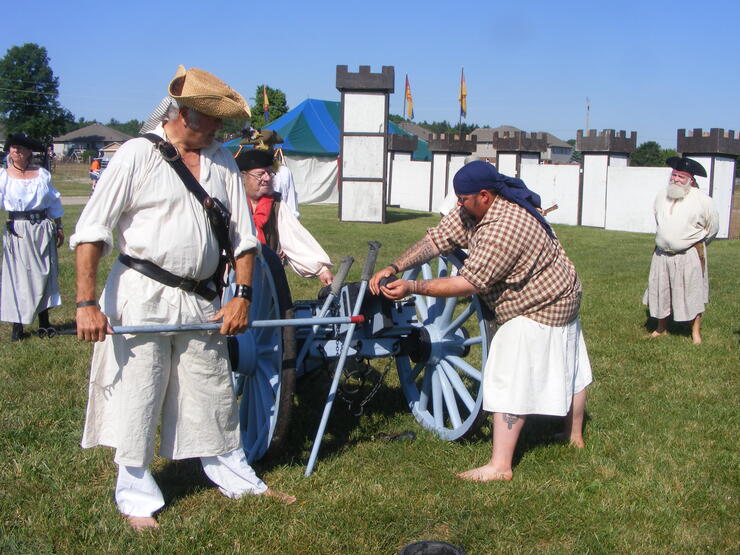In this vivid color photograph, the scene is set under a bright, clear blue sky with no clouds and a vibrant green grassy field beneath. The focal point is a group of people engaged in a medieval or Renaissance reenactment. Prominently, there are three men participating in what appears to be the loading of a blue and black cannon. 

The man on the right, who is overweight and tattooed, wears a blue headscarf, a cream and brown checkered shirt, and a white kilt. He has tattoos on one arm and is in the process of handling a baby blue wheelbarrow. To his left stands another man in a straw hat, dressed in a loose-fitting linen button-up shirt and wide-legged linen pants. A third man, sporting a pirate hat and a long white beard, is visible in the background wearing all white. 

Additionally, there's a woman dressed in attire reminiscent of a female pirate, adding to the historical ambiance. Behind them, a make-believe cardboard castle structure and a white building that resembles a castle provide a fitting backdrop, enhancing the overall medieval atmosphere of the scene.